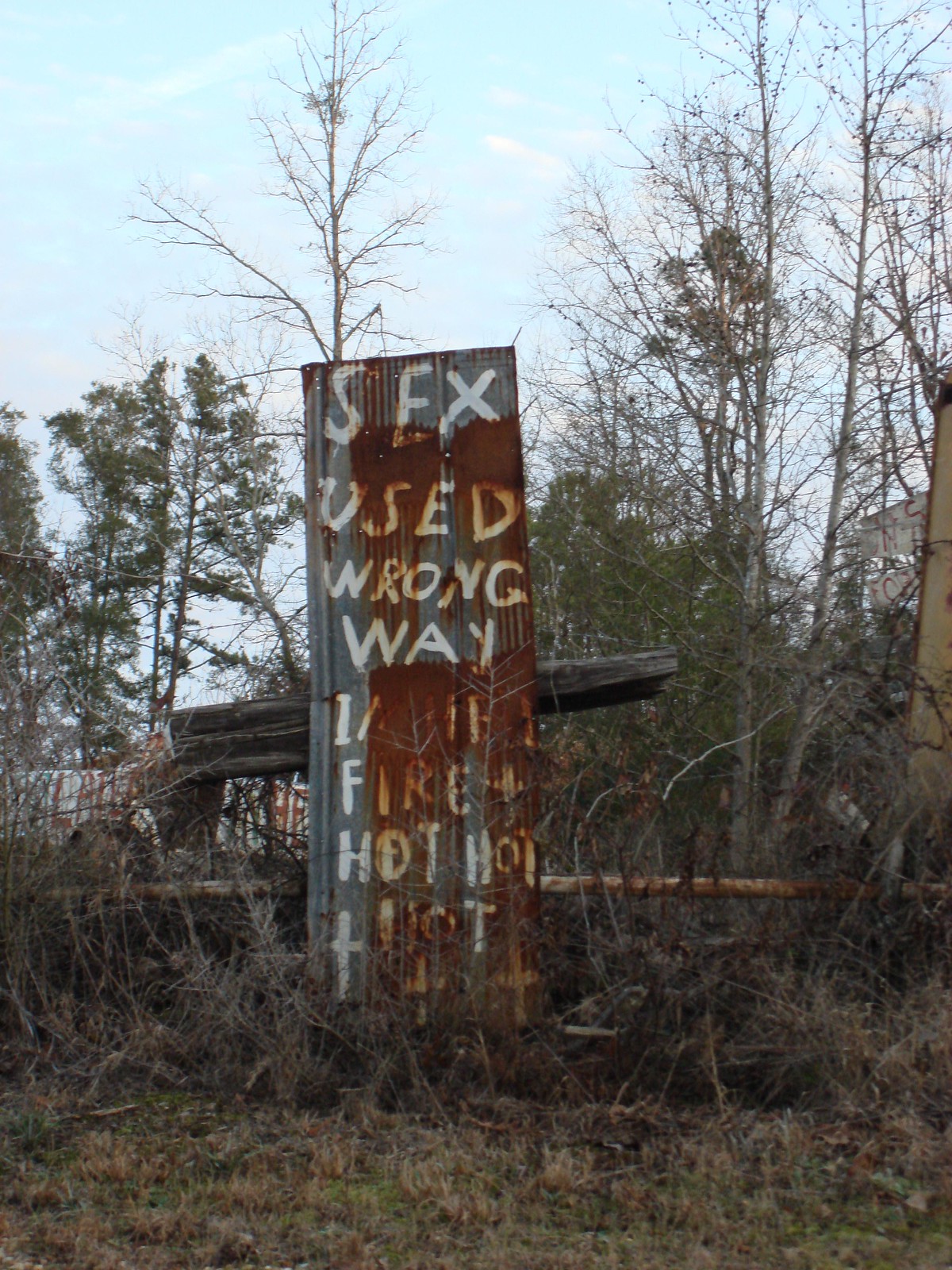An image features a rustic, weather-beaten metal sign, reminiscent of something you'd find in a junkyard. The immediate surroundings are overgrown and neglected, with a clutter of fallen trees and scattered wood pieces. The sign itself stands tall, fashioned from a rusty, vertically ribbed metal sheet, likely part of an old shed's siding. Faded and partially obscured by rust, the sign's legible text reads: "Sex used wrong way," followed by an indecipherable section, then concluding with the bold and repetitive "Hot, hot, hot." The scene evokes a sense of abandonment and decay, juxtaposed with the provocative and puzzling message of the sign.